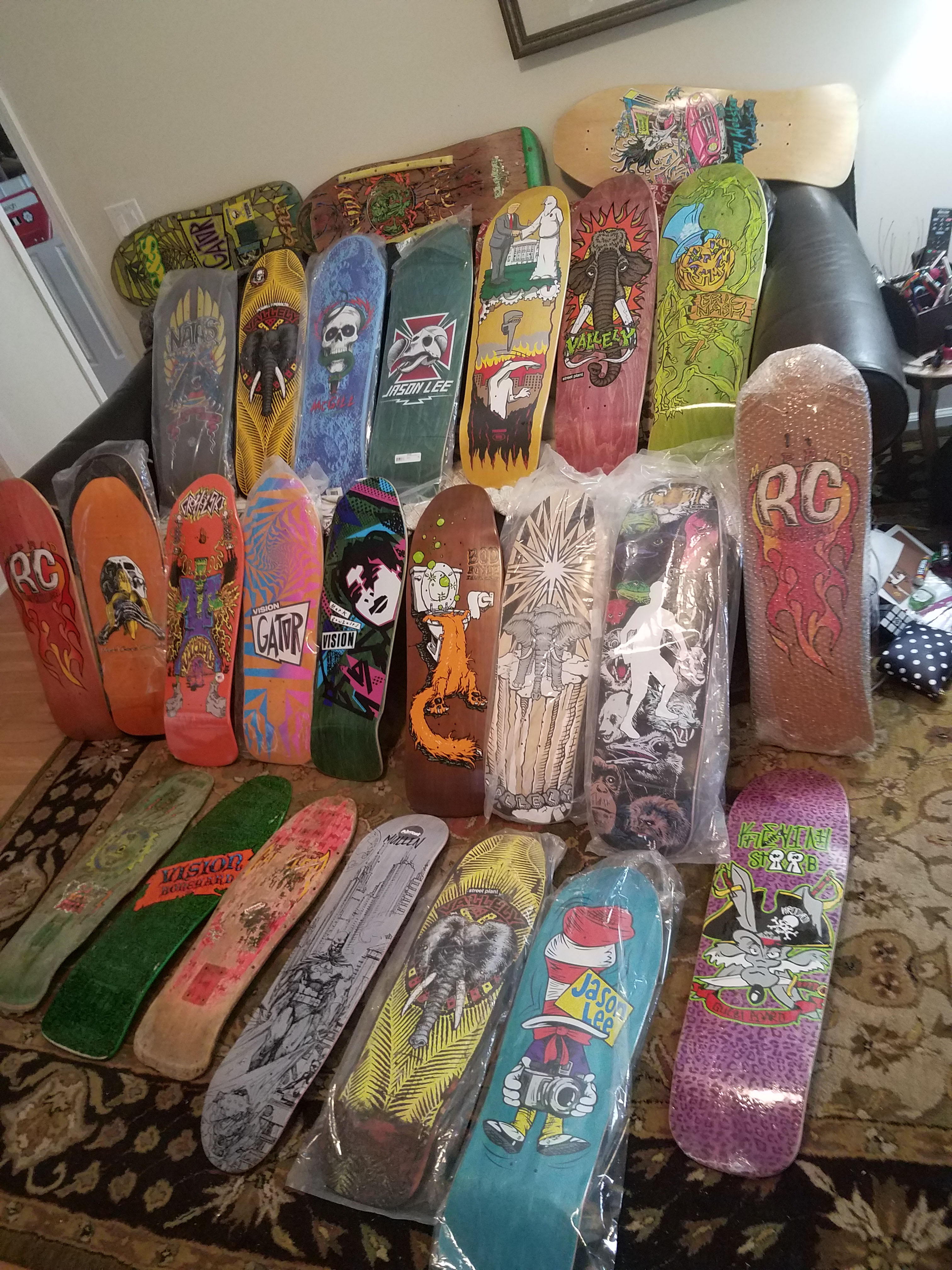This photograph captures a vibrant collection of skateboards inside a living room. Each skateboard, stripped of wheels and trucks, showcases unique and brightly colored graphics, ranging from skulls and elephants to cartoon characters. The boards are meticulously arranged in rows: three lean against a white wall above the back of a black leather couch, seven rest on the couch's seat, nine stand upright against the front of the sofa, and seven more lie flat on a tan, black, and blue Persian-style rug. Some of the skateboards are wrapped in plastic cellophane bags, adding a glossy texture to the scene. In the living room, a nearby table holds a basket with various items, including a TV remote, against cream-colored walls. The overall aesthetic is a mixture of organized chaos and artistry, reflecting the vibrant and diverse nature of the skateboard graphics.